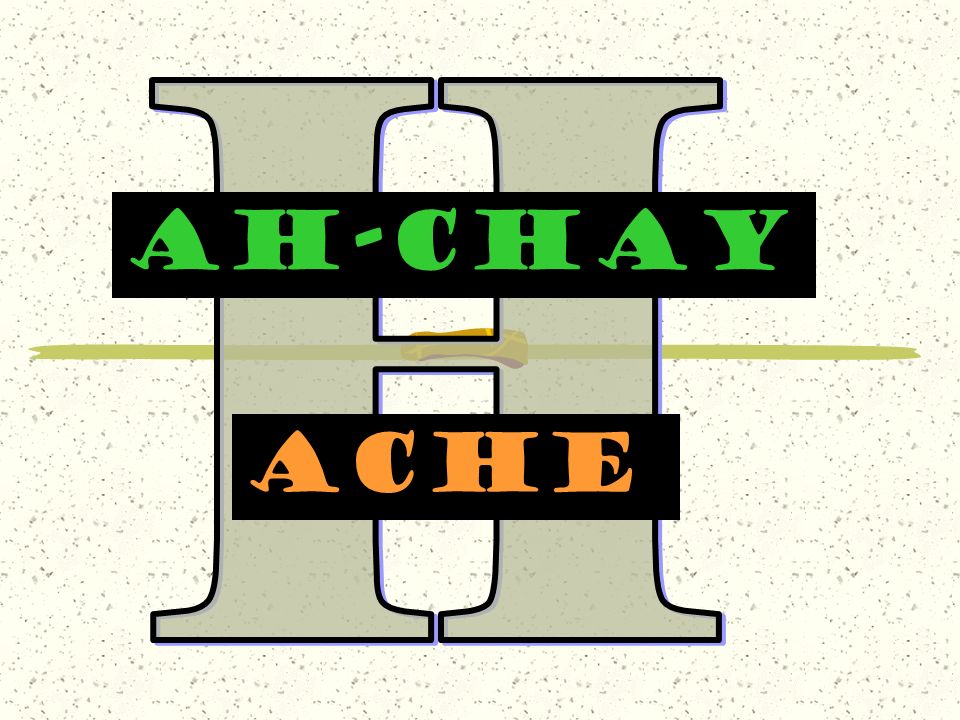The image features a central, large, grayish-green letter "H," bordered with a thick, dark black outline, situated against a light off-white background speckled with fine green grains. The image has a horizontal orientation, being longer left to right. A light green stripe runs horizontally through the center of the letter "H," extending almost from edge to edge of the image. Positioned across the top half of the "H" is a black rectangular bar containing green block letters spelling "AH-CHAY." A matching black bar is located across the bottom half of the "H," with orange block letters spelling "ACHE." The letter "H" is semi-transparent, giving it a slightly see-through appearance, and the combined elements suggest it could be a logo or an icon, possibly related to a college or organization.